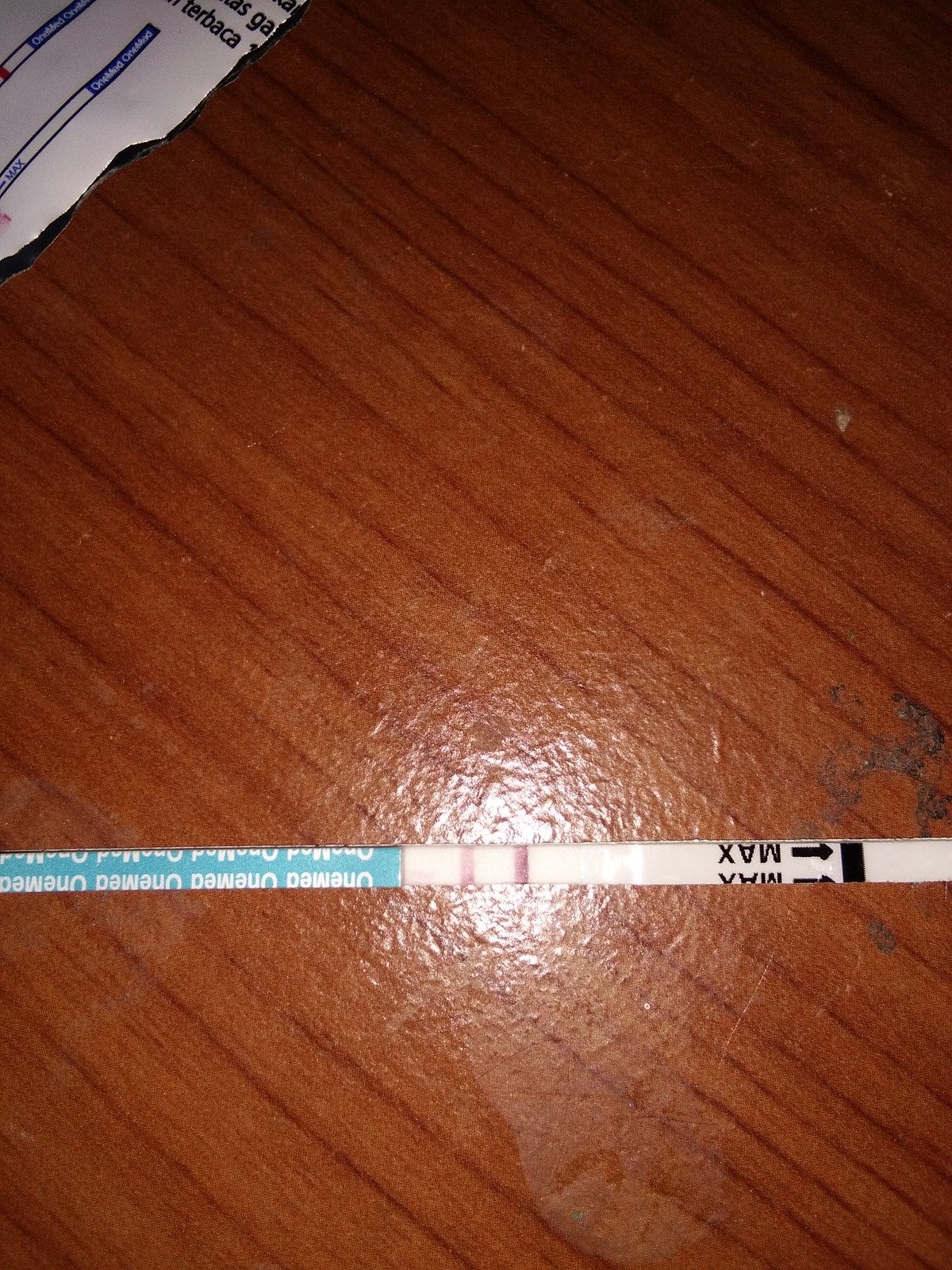An aerial view captures a rectangular section of a wooden floor characterized by its reddish-orange undertones and visible grain patterns marked by darker lines. On the right side of the image, near the middle, a small clump of dirt is noticeable. A light source creates a glare on the floor, illuminating a significant smudge nearby. In the upper left corner, a torn piece of white paper is seen, possibly displaying test instructions. At the center of the composition lies a white test strip, most likely a pregnancy or ovulation test, featuring two pink lines and a blue strip at its bottom.